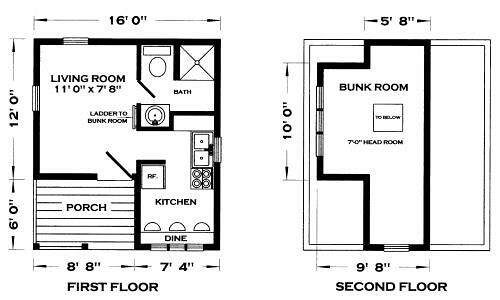This blueprint showcases the detailed layout of a two-story house. The left side of the blueprint outlines the first floor, while the right side displays the second floor. 

Starting at the bottom of the image, the first floor features a porch that serves as the main entrance to the house. Upon entering through the porch, you are welcomed into a spacious living room. Adjacent to the living room is a ladder that provides access to a bunk room situated on the second floor.

In the top right corner of the first floor, there is a bathroom equipped with essential amenities, including a shower, toilet, and sink. Moving back to the porch entry, the first door on the right leads to the kitchen. The kitchen is furnished with a small dining table and dining bench, a cooker, and likely a double sink. The kitchen seamlessly flows into the living room, creating an open-plan design devoid of any doors.

The right side of the blueprint details the second-floor layout, specifically the bunk room. The bunk room's dimensions and shape are irregular, indicating it doesn't occupy the entire footprint of the first floor. Access between the bunk room and the living room downstairs is facilitated by the ladder.

This blueprint provides a comprehensive overview of the house's structure, highlighting the thoughtful spatial arrangement and functional design elements over two floors.